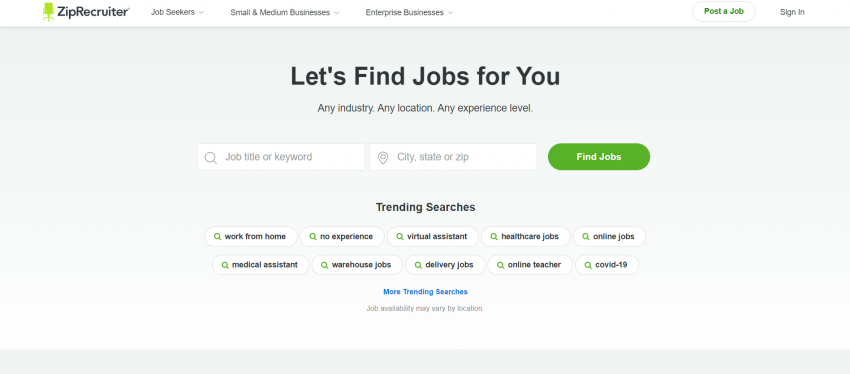This is a detailed caption for an image of the ZipRecruiter "Find a Job" webpage, framed to provide a clear and comprehensive description:

The image features a cropped screenshot of the ZipRecruiter "Find a Job" page. Dominating the top portion of the image is a white header that spans the width of the page. On the far left of this header, the recognizable ZipRecruiter logo is prominently displayed. Adjacent to the logo on the right are three primary categories: "Job Seekers," "Small and Medium Businesses," and "Enterprise Business," each accompanied by a drop-down menu for further navigation options. Positioned on the far right of the header are two circular icons. The first is a green button marked "Post a Job," and the second is a gray button labeled "Sign In."

The body of the webpage has a gradient background that transitions from gray at the top to white at the bottom, adding a visual depth to the interface. At the very top of this section, centered on the page, is the motivational heading, "Let's Find Jobs for You," rendered in a large, clear font. Below this heading, a subtext reads, "Any Industry, Any Location, Any Experience Level," in small black letters, summing up the website's inclusive job search promise.

Further down, the user is presented with a search interface consisting of two boxes. The first box prompts the user to input a "Job Title or Keyword," while the second box, located to the right, is for specifying a "City, State, or Zip." Completing this search interface is a green oval button to the far right, bearing the command "Find Jobs" in small white font, designed to initiate the job search process.

Centered just below the search interface, the text "Trending Searches" is boldly displayed in black font, capturing the user's attention. Underneath this heading are two rows of bubble-shaped suggestion buttons. Each bubble features a small magnifying glass icon on the right side and provides popular search terms such as "Work from Home," "No Experience," "Virtual Assistant," "Healthcare Jobs," and "Online Jobs." These suggested searches aim to guide users toward trending job categories.

This detailed description offers a comprehensive overview of the webpage's layout, elements, and functionalities, demonstrating the user-centric design of the ZipRecruiter platform.